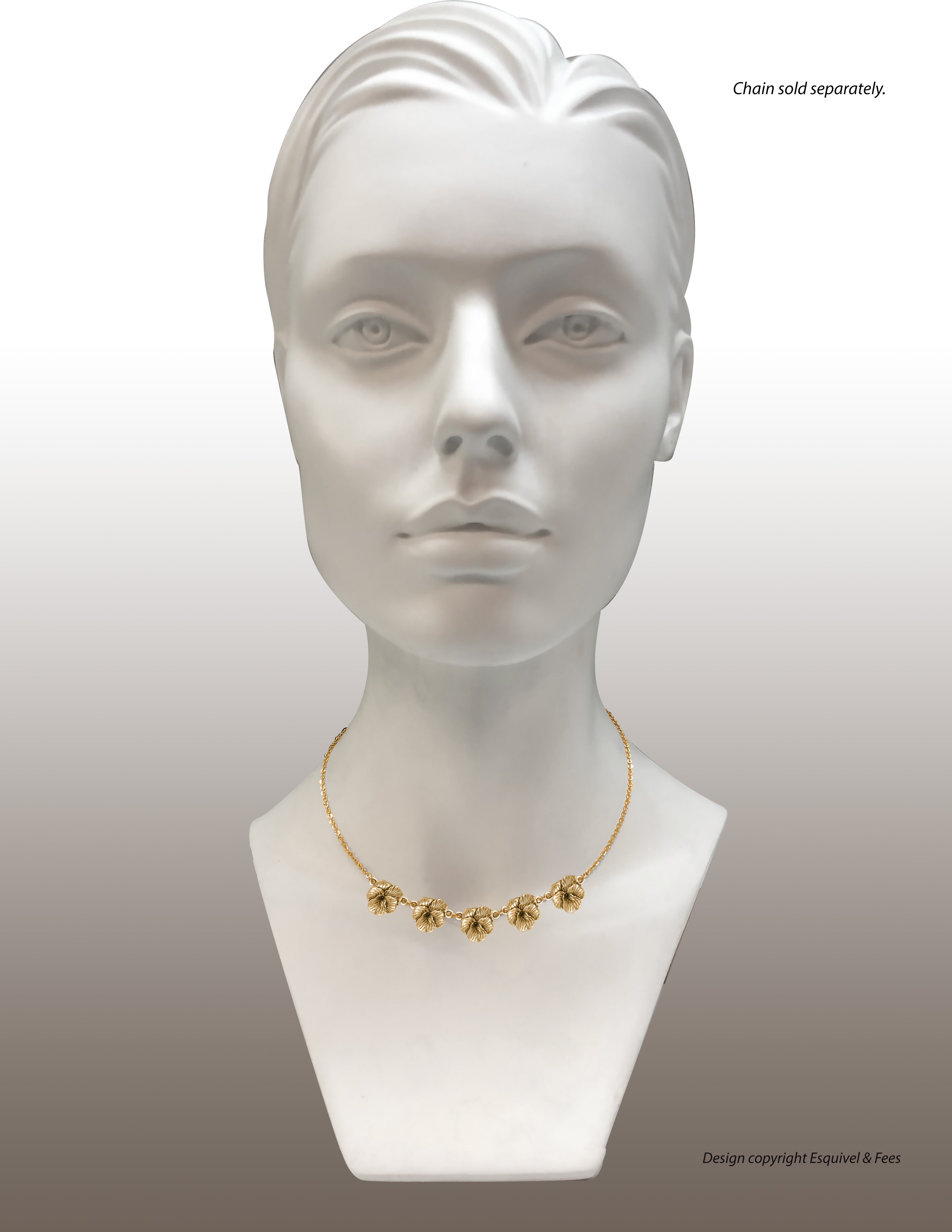This photograph depicts a white, ceramic female mannequin head, commonly seen in department store jewelry sections. The minimalist composition features a gradient background that transitions from a bright white at the top to a darker grayish-brown at the bottom. The mannequin showcases a brushed-back hairstyle and detailed facial features including prominent eyes, nose, and lips. Around its neck is a thin, dainty gold box chain adorned with five small, golden floral charms resembling hibiscus flowers. The chain is clearly marked as "sold separately" in black text at the top right corner of the image, while the bottom right corner bears the inscription "Design, copyright, Esquivel, and fees."